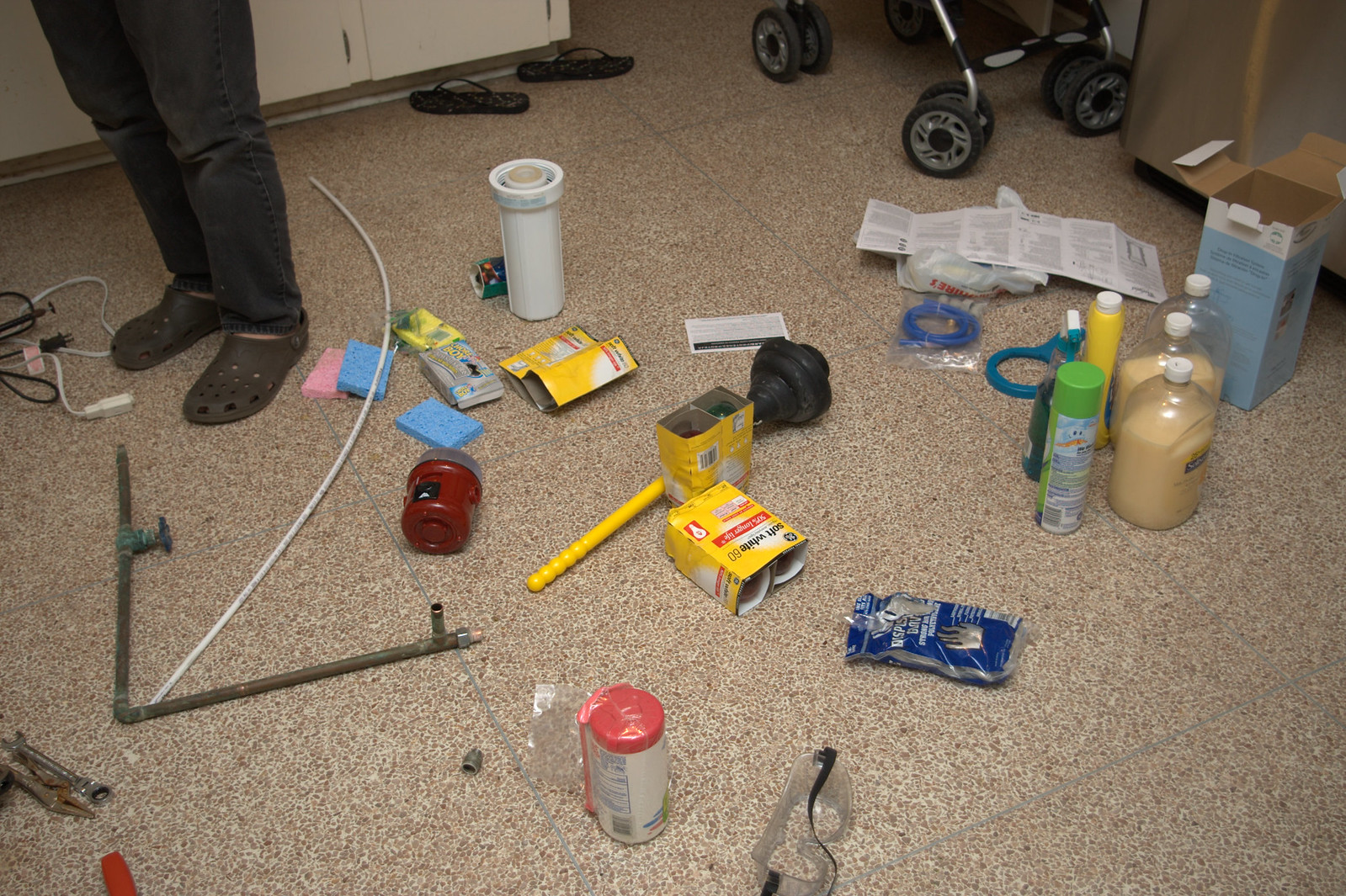A bustling indoor kitchen scene is captured in this image. In the background, a stroller is visible, suggesting a family-oriented environment. The kitchen features sleek white cabinets that contrast with the cluttered floor. A pair of flip flops is casually left on the large, stone-like tiled floor, which appears to be grouted. Standing in the midst of this organized chaos is a person wearing gray Crocs and black jeans. Scattered around are various items that indicate home maintenance activity: light bulbs, an air filter, a plunger, cleaning products, hand soaps, a piece of pipe, tubing, tools, goggles, plastic gloves, sponges, and electrical cords. It seems these items were hastily pulled out of a cabinet to facilitate some repair work on the pipes beneath. The person in Crocs remains stationary, their actions concealed from view, adding a sense of anticipation to the scene. The overall ambiance is one of practical chaos, capturing a moment of maintenance and repair in a lived-in home.